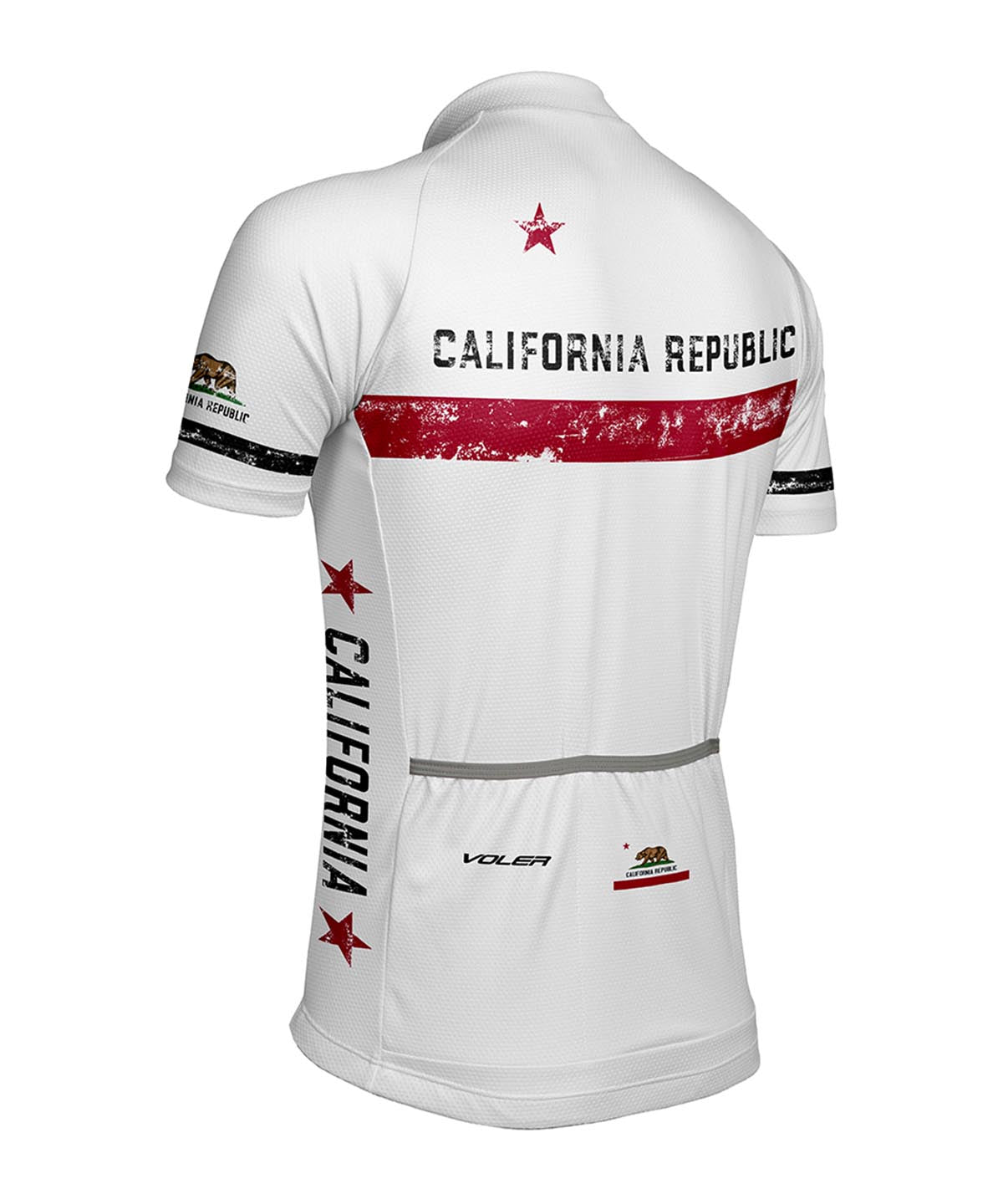In the image, there is a short-sleeve shirt that appears to be part of a soccer team uniform. The shirt is predominantly made of cotton fabric, showcasing a comfortable and breathable design. It is displayed on a mannequin, although the mannequin itself is not visible; the shirt's form suggests it is being worn. The shirt is photographed from the back, revealing the left side angled slightly towards the upper left of the image. Across the upper back of the shirt, the words "California Republic" are prominently printed, accompanied by a red horizontal bar below the text. The detailed display and the shirt's presentation provide a clear view of the design and branding, indicating its function as a sports uniform.